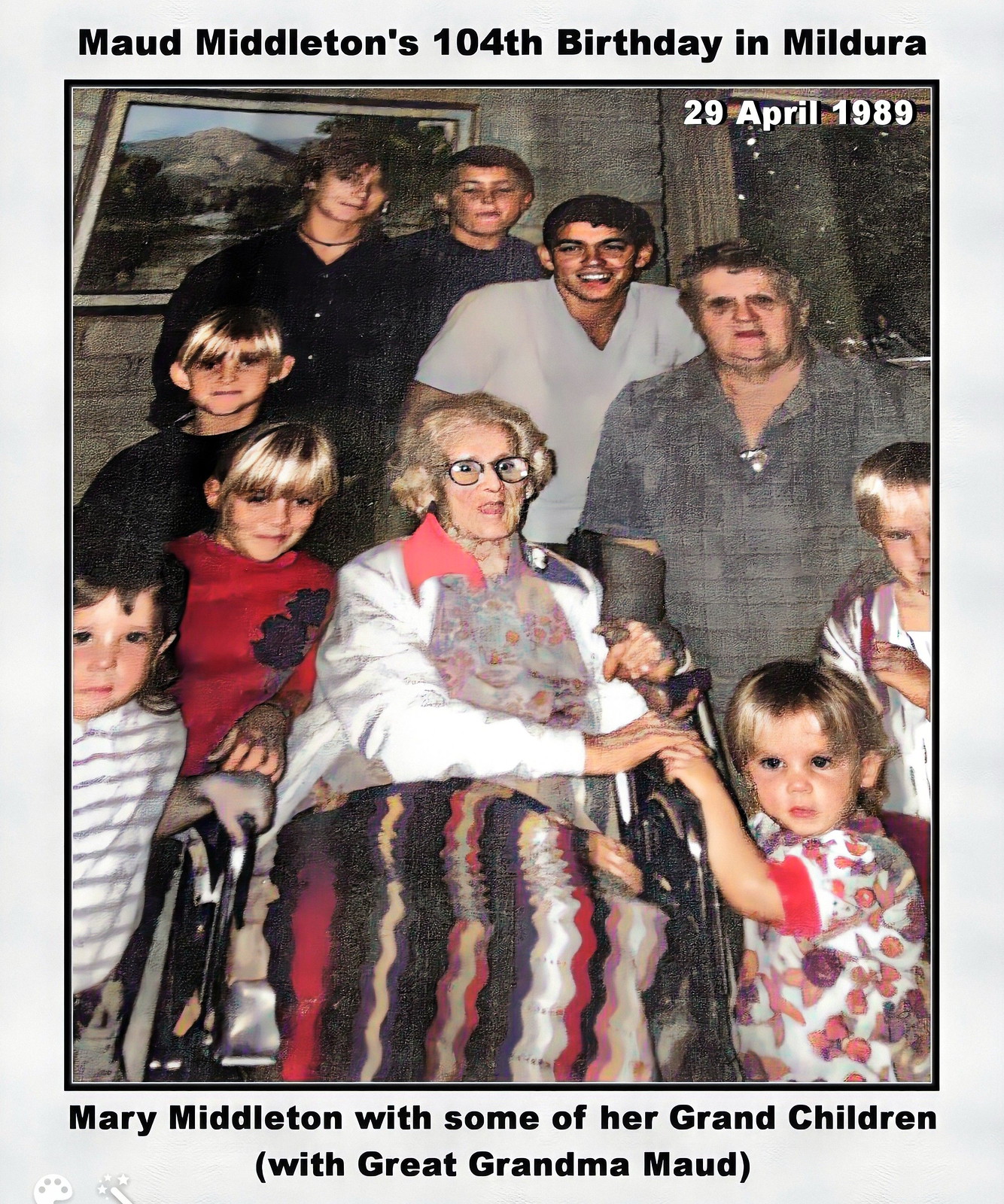The image is a printed photo framed by a gray border, dated 29 April 1989, and captioned at the top with "Maude Middleton's 104th Birthday in Mildura." The bottom caption reads, "Mary Middleton with some of her grandchildren, with great-grandma Maude." Maude, in a white shirt and a striped blanket on her lap, is seated in a wheelchair at the center of the photo. She has glasses and short, light-colored hair, and her mouth is slightly open. Surrounding her are a group of children: four with blonde hair and one with brown hair. To her left and right, there are children with differing heights and hair colors, including one in a white striped shirt. Behind Maude stand several teenagers and possibly an adult male. They all pose amid an indoor setting featuring drapes, a brick wall, and a painting in the background. Some subjects smile while others look directly at the camera. The scene suggests a family gathering to celebrate Maude's significant milestone birthday.